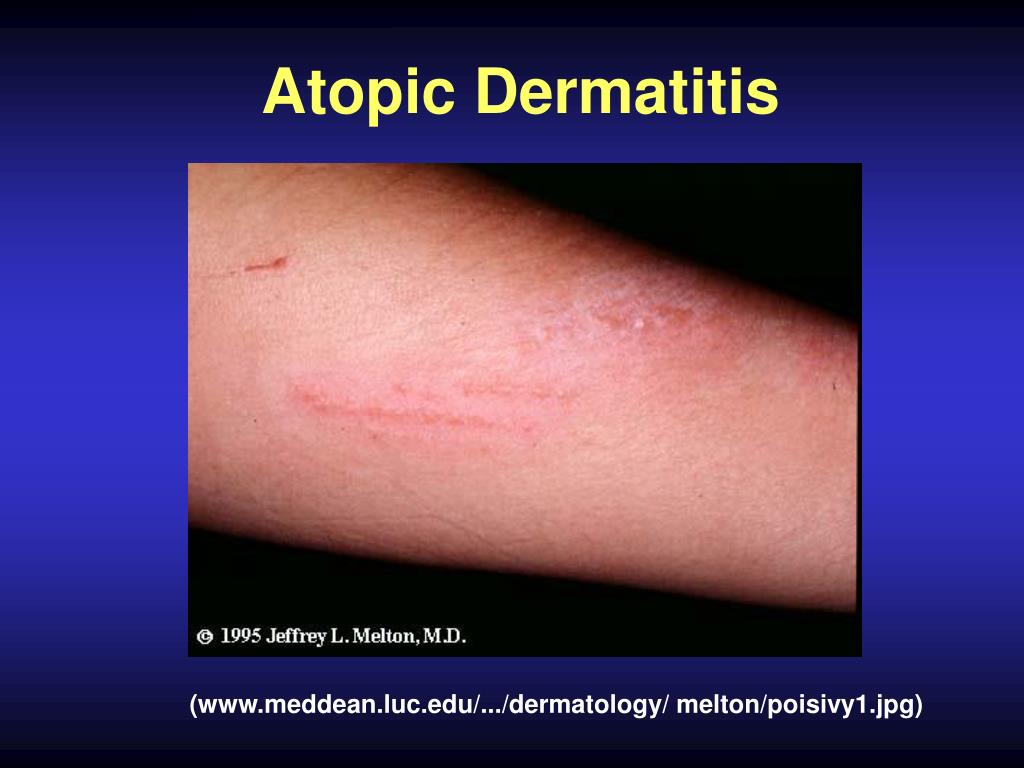The image appears to be a detailed slide from a medical journal or educational presentation, depicting a case of atopic dermatitis. The main focus is a photograph of a white person's forearm, prominently showing a dry, itchy, red rash, characterized by red, white, and pink scars. The background of the slide features a dark blue to black horizontal border, with the words "Atopic Dermatitis" displayed prominently in yellow across the top. The forearm appears to be resting on a black surface, and the rash runs diagonally across it. The image is credited to Jeffrey L. Melton, M.D., 1995, and at the bottom, it provides a website link: www.meddean.luc.edu/.../dermatology/melton/poisoniv1.jpg. The slide is straightforward yet comprehensive, indicative of its purpose as an educational resource.